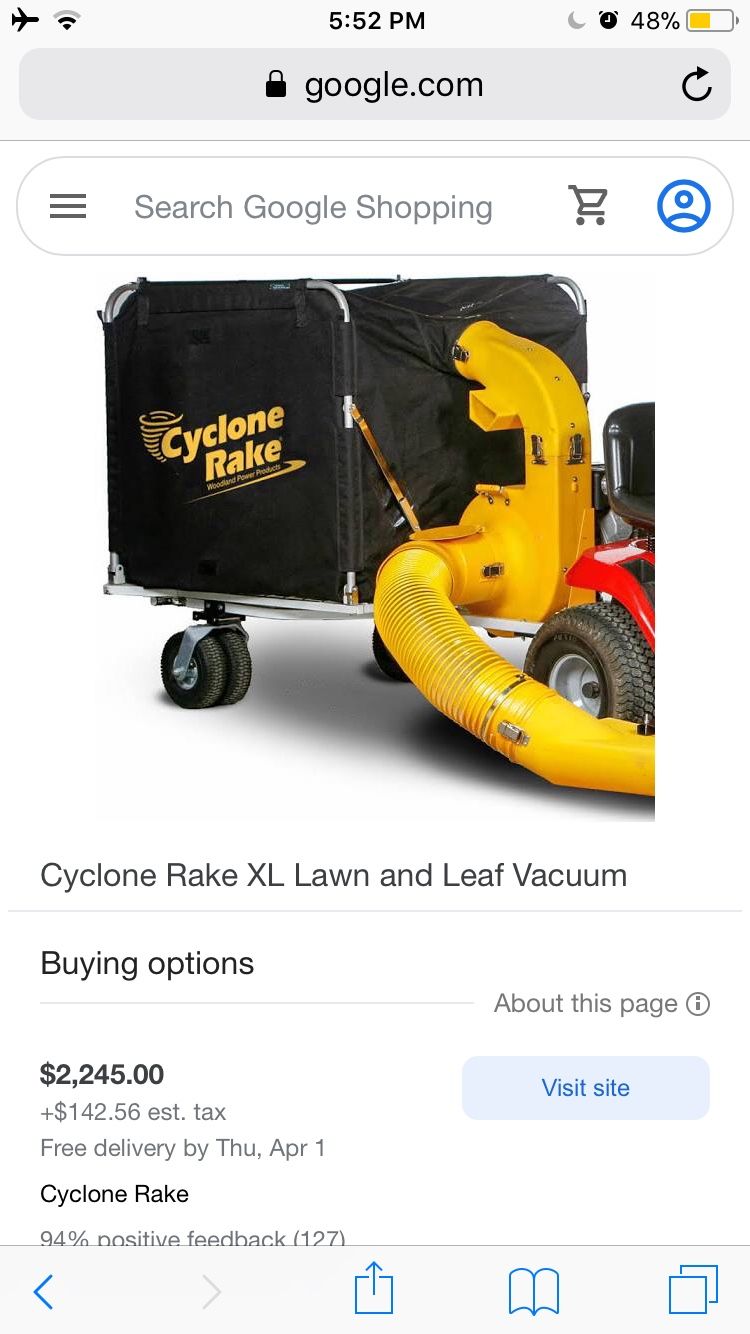The image depicts a webpage displayed on a smartphone, with the URL "goku.com" clearly visible. The top tab features a search bar labeled "Search GOKU SHOPPING," flanked on the left by a menu icon consisting of three black horizontal lines and on the right by a grey cart icon and a blue profile icon. Above these icons in the browser, there is a black refresh icon.

Below the search bar, the central focus is on a black and yellow device with wheels. The wheels are black, and the body of the device prominently displays the text "CYCLONE RAKE" in yellow. Beneath this, in smaller text, it reads "CYCLONE RAKE XL LOUNGE & LIFT VACUUM BUYING OPTIONS." The price is listed as "$2,245 plus $142.56 estimated tax," with a note indicating "free delivery by Thursday, April 1." The product boasts "94% positive feedback" from 127 reviews.

On the right side of the product description, there is a blue button labeled "Visit site." Above this button, grey text reads "About this page." The entire webpage is set against a white background.